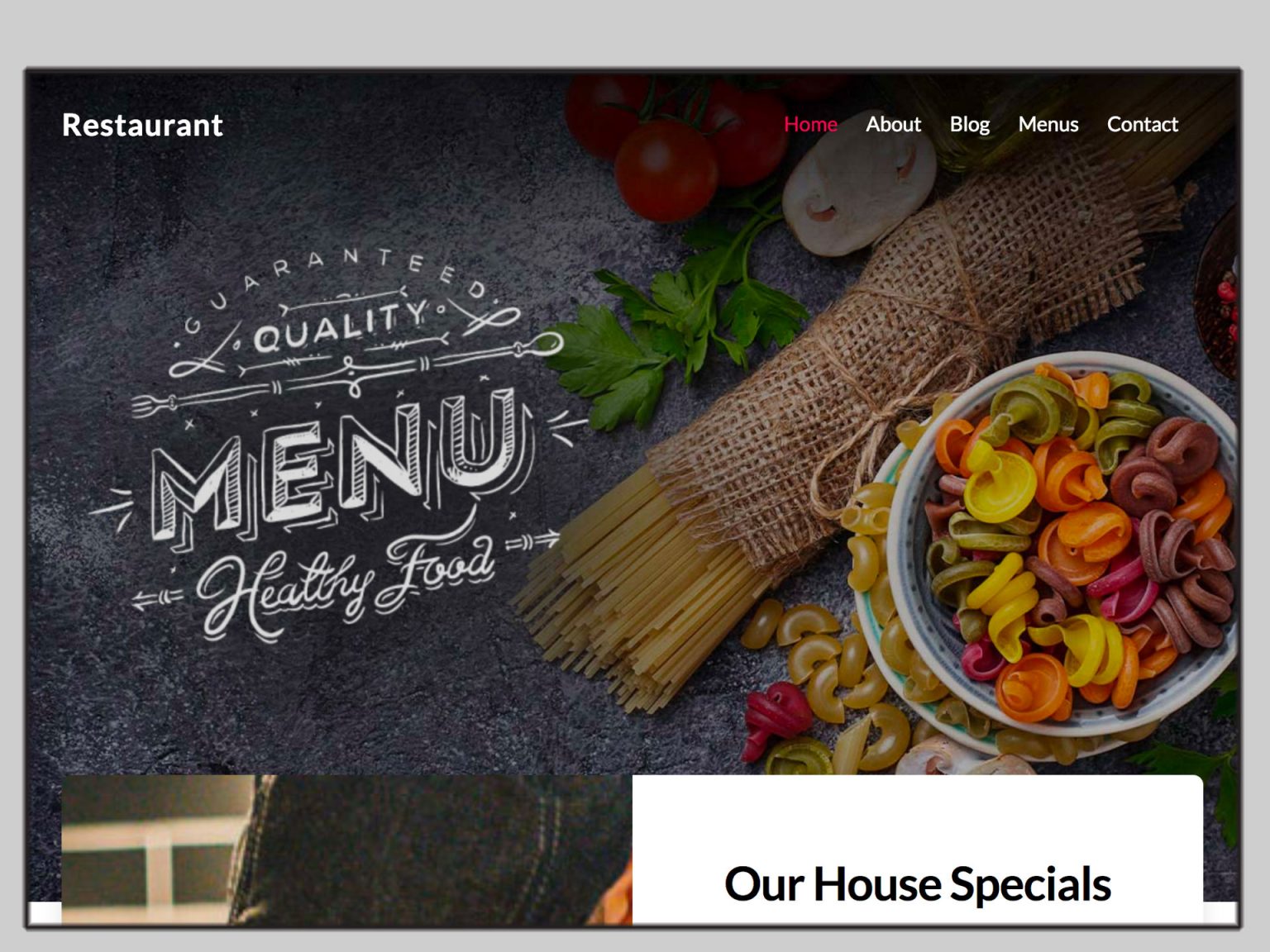"Indulge in Quality Cuisine: This enticing advertisement showcases a sophisticated restaurant experience. At the top left, the word 'Restaurant' is prominently displayed in elegant white text. To the top right, a navigational menu with tabs such as Home, About, Blog, Menus, and Conduct can be seen; all are written in white except for 'Home,' which is highlighted in red.

Dominating the left-center, a cluster of white text proudly proclaims 'Guaranteed Quality, Menu, Health, Food,' emphasizing the restaurant's commitment to excellence. On the bottom right, a notable black text on a white background announces 'Our House Specials.'

The backdrop of the advertisement features an inviting gray surface abundantly adorned with delectable food items. A vibrant green plant spruces up the display, complemented by a generous serving of yellow spaghetti and a medley of macarons in varying hues—brown, red, pink, yellow, dark brown, and dark green. These colorful macarons, some placed in a bowl on the right, are artfully presented in a white and gray bowl with a pristine white and green plate below.

Adding to the visual feast, a richly red tomato sits at the upper part, perfectly ripe, while a garlic bulb, gleaming white, takes center stage, completing this appetizing tableau designed to entice and delight food enthusiasts."